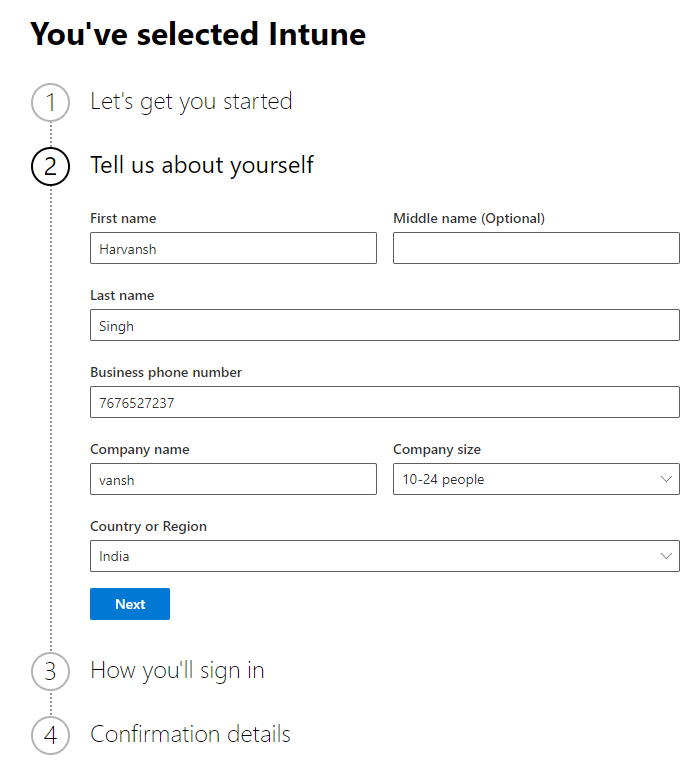A detailed caption for the described image could be:

"This screenshot shows the initial setup page of a website, where a user is required to input their personal and professional information. The interface is predominantly white with black text, providing a clean and straightforward look. At the very top, the text reads 'You've selected Intune,' followed by a welcoming message in a numbered sequence. 

Step one is labeled 'Let's get you started,' and step two prompts the user to 'Tell us about yourself.' In the user input fields below, the first name 'Harvanish' (spelled H-A-R-V-A-N-S-H) is entered. The middle name is listed as optional and has been left blank. The last name entered is 'Singh' (spelled S-I-N-G-H). 

The next field requires a business phone number, which is filled with '767-652-7237.' The subsequent field asks for the company name, where 'Vansh' (spelled V-A-N-S-H) has been entered. The form also includes the company size, which is indicated as '10 to 24 people,' and the company’s region, specified as 'India.'

Lastly, there is a visible 'Next' button that likely leads to further steps, including how the user will sign in and confirm their details."